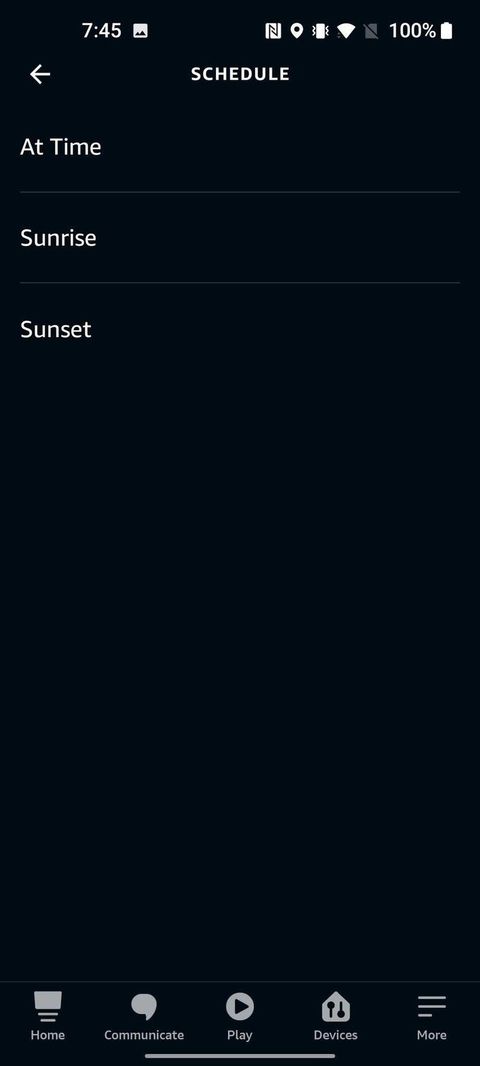The image is a screenshot of a phone screen with a black background. In the upper left-hand corner, the time is displayed as 7:45, with a colon separating the hour and minute. Next to the time, there is a series of icons including a photo icon, NF connection, map connection, a phone with two bars on either side, and a fan icon. Following these icons is a rectangular box with a line through it. Adjacent to this, it indicates 100% battery life with a vertical white battery icon.

Below the icon bar, aligned to the left, there is a left arrow icon. The word “SCHEDULE” is prominently displayed in all caps. Below this, it says “At Time.” A horizontal line runs from left to right under it. Below the line, the words “Sunrise” and “Sunset” are listed sequentially.

At the very bottom of the screen, there are five icons spaced evenly: The first icon, labeled “Home,” has a rectangular shape with two bars beneath it. The second icon is labeled “Communicate,” marked by a speech bubble resembling those seen in cartoons. The third icon labeled “Play” features a white circle with a black right-facing arrow. The fourth icon, labeled “Devices,” shows a house with two sliders (one slider positioned upwards and one downwards). The fifth and final icon is labeled “More,” featuring two equal-sized bars with one bar slightly shorter than the other.